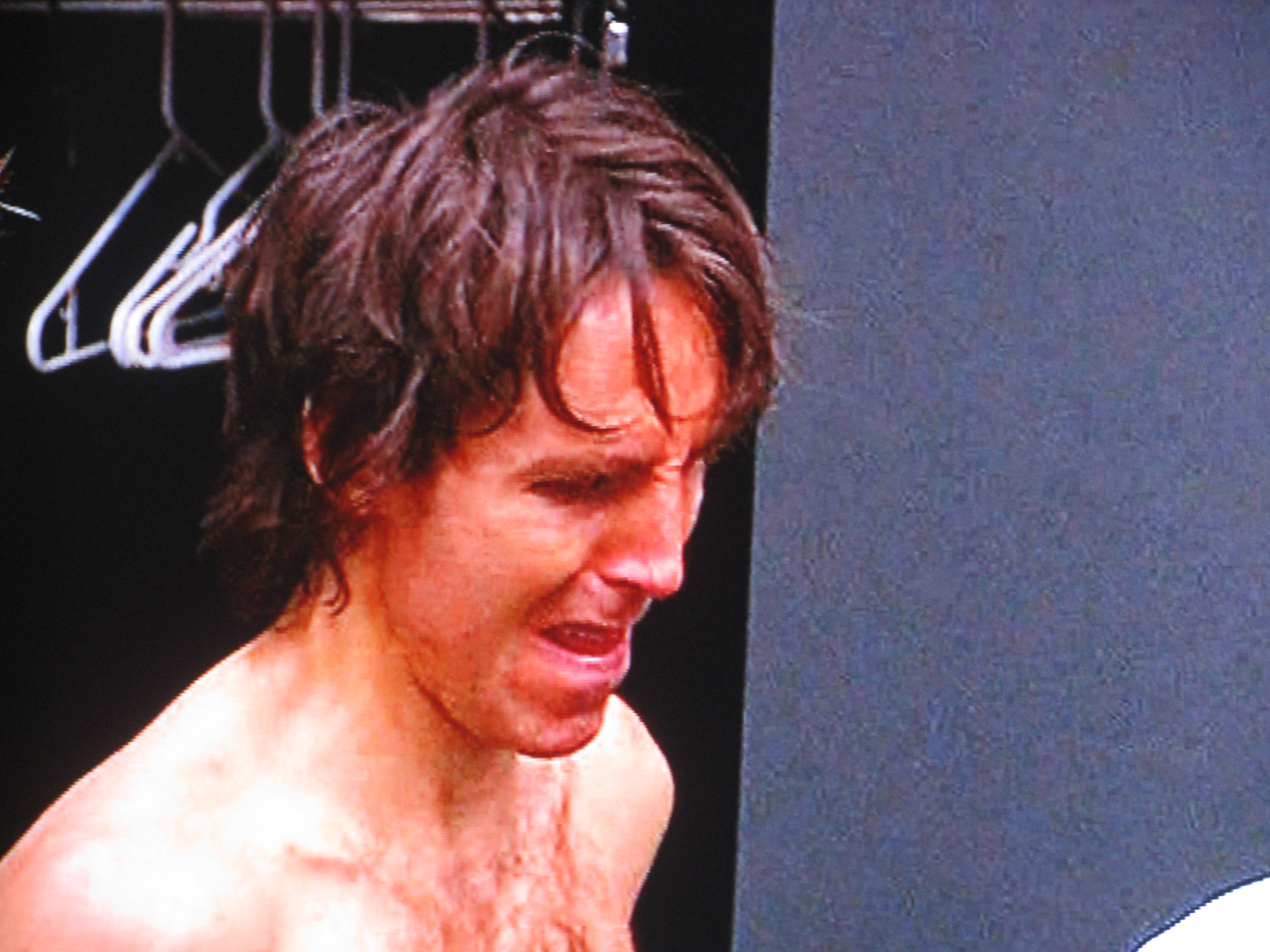In the center of this indoor image, a shirtless young man with moderately long, loose brown hair is prominently featured. The man’s eyes are tightly scrunched, his lips parted, and his expression conveys significant discomfort or pain, potentially indicating he just finished a fight or received bad news. His thin frame, with pronounced shoulders, is positioned directly in the center of the picture. Behind him, the setting appears to be a dressing room, with a black and blue wall and white hangers hanging to the left, above an area that looks like a closet. The background, displayed off to the right, shows a bit of a wall. The colors in the image are predominantly black, white, tan, brown, gray, and silver, and the man appears to have a mouthguard or similar item in his mouth.